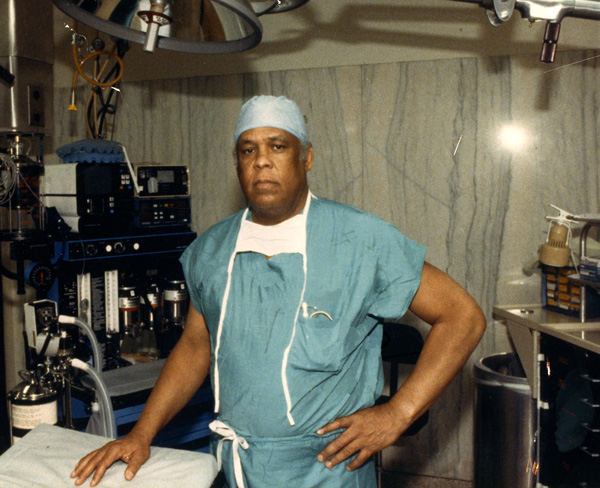The image depicts a 50-year-old black surgeon standing in the middle of an old-fashioned surgical room. He is dressed in teal blue scrubs, which include a blue surgical cap and a white surgical mask hanging around his neck. Notably, the surgeon has visible white sideburns and strikes a composed stance with his left hand resting on a white gurney and his right hand on his waist. The scrubs feature long white ties, and the matching pants are cinched at the waist with a white tie. The background reveals a white marble wall with blue vertical stripes, partially obscured by various pieces of surgical machinery. To the surgeon's left are some containers within a mostly black machine, along with an oxygen tank. Toward the bottom right corner, a waste basket and a cabinet are visible. Additionally, the upper right corner of the image shows part of a medical machine and a connected pipe, while bright, unlit medical lights with silver outlines loom above the scene.